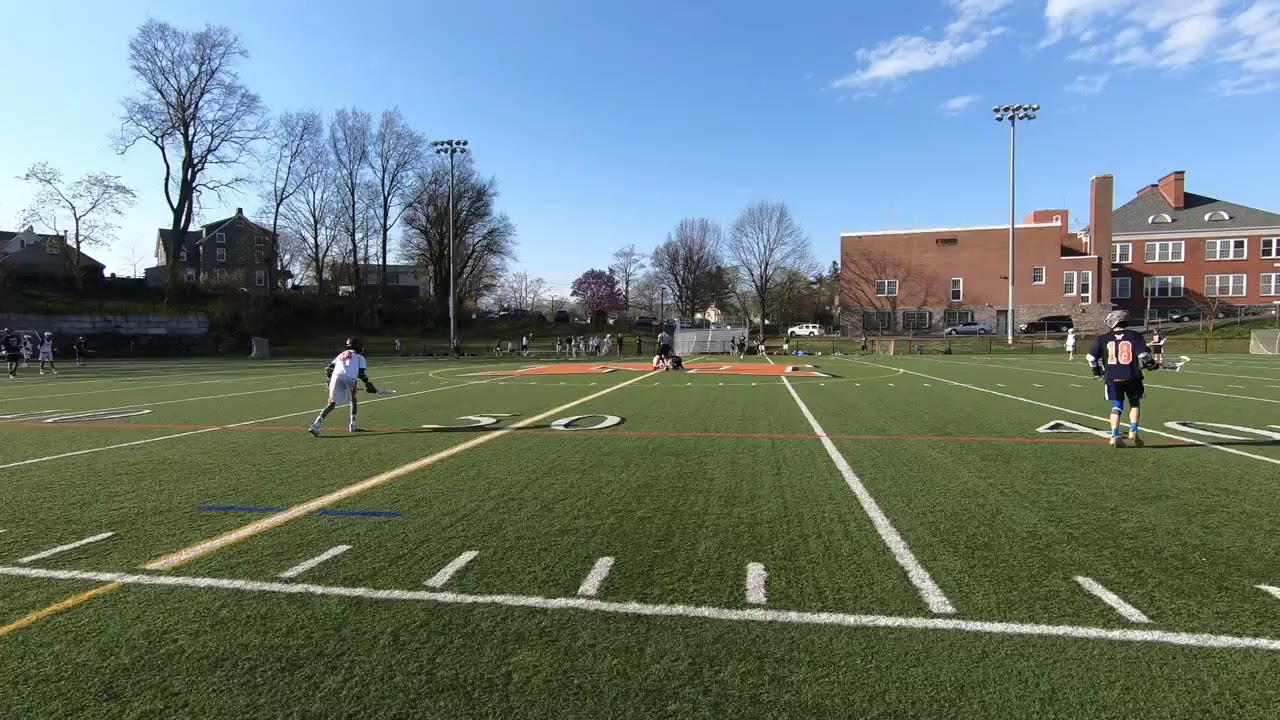The image depicts a group of teenage or adult men playing lacrosse on a green field, marked with numerous white horizontal lines and a vertical line near the bottom, intersected by smaller vertical lines. Two players are prominently featured: one on the left wearing a white jersey, and another on the right sporting a black jersey with the number 10 on his back. In the background, a netted goal with a ledge is visible, with other players congregated around it. Surrounding the field, there are tall trees, a brown building with a triangular roof and chimney on the right, and additional structures including brick houses, an office building, and roads lined with small cars. The scene is set under a clear blue sky, likely around midday. Additionally, a large orange "M" is visible in the middle of the field, suggesting the location might be a college or school football field.